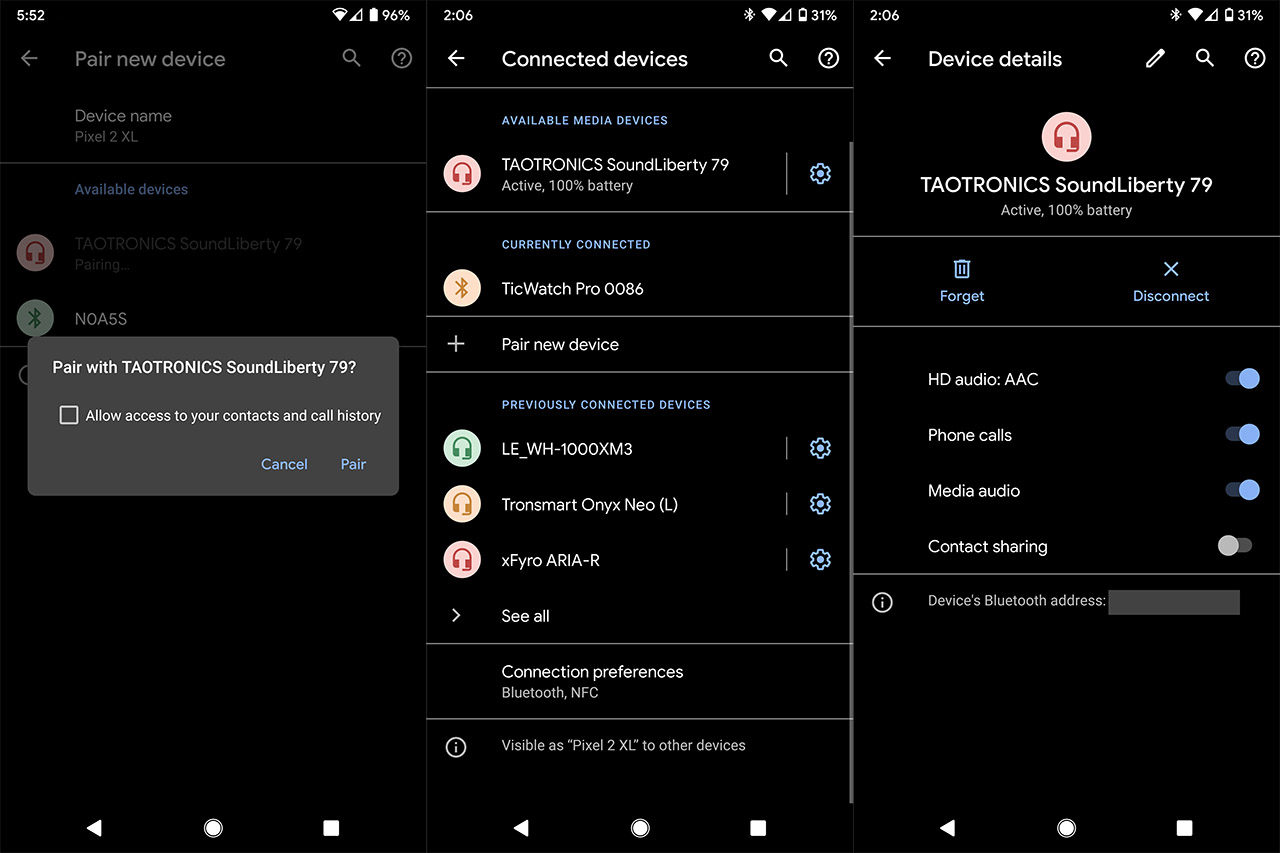The image consists of three side-by-side smartphone screenshots displayed in dark mode, featuring interfaces predominantly in black with white text. Each screenshot presents a different screen within a Bluetooth and device connectivity setting.

### First Screenshot:
- **Top Bar:** Displays the time at 5:52, signal strength, Wi-Fi status, and battery life at 96% in the upper right corner.
- **Main Section:** 
  - A heading "Pair new device" in gray font with an arrow pointing to the left.
  - Icons for a magnifying glass (search function) and a question mark (help) on the right.
- **Content Below Main Heading:**
  - "Device name" heading followed by "Available devices" list.
  - A prominent pop-up in the forefront: 
    - "Pair with Teotronic Sound Liberty 79".
    - An option box to allow access to contacts and call history.
    - Buttons labeled "Cancel" and "Pair" in light blue.

### Second Screenshot:
- **Top Bar:** Displays "Connected devices" in white text, with icons for a magnifying glass and help on the right.
- **Main Content:**
  - "Available media devices" in light blue, with "Teotronic Sound Liberty 79" listed in white text and a gear icon on the right.
  - "Currently connected" device labeled "TikTok Pro".
  - "Pair new device" section, followed by "Previously connected devices" in blue font.
  - List of four previously connected devices.

### Third Screenshot:
- **Center of Screen:** Features a circle with a red headset icon.
- **Below Icon:**
  - Text stating "Teotronic Sound Liberty 79".
  - Two buttons labeled "Forget" and "Disconnect".
- **Audio Options Section:**
  - Four audio options: "HD audio," "Phone calls," "Media audio," and "Contact sharing".
  - Radio buttons beside options, the first three turned on, and the fourth ("Contact sharing") turned off.

The detailed descriptions provide a comprehensive understanding of each screenshot's interface, emphasizing the Bluetooth pairing and device management functionalities across the three screens.